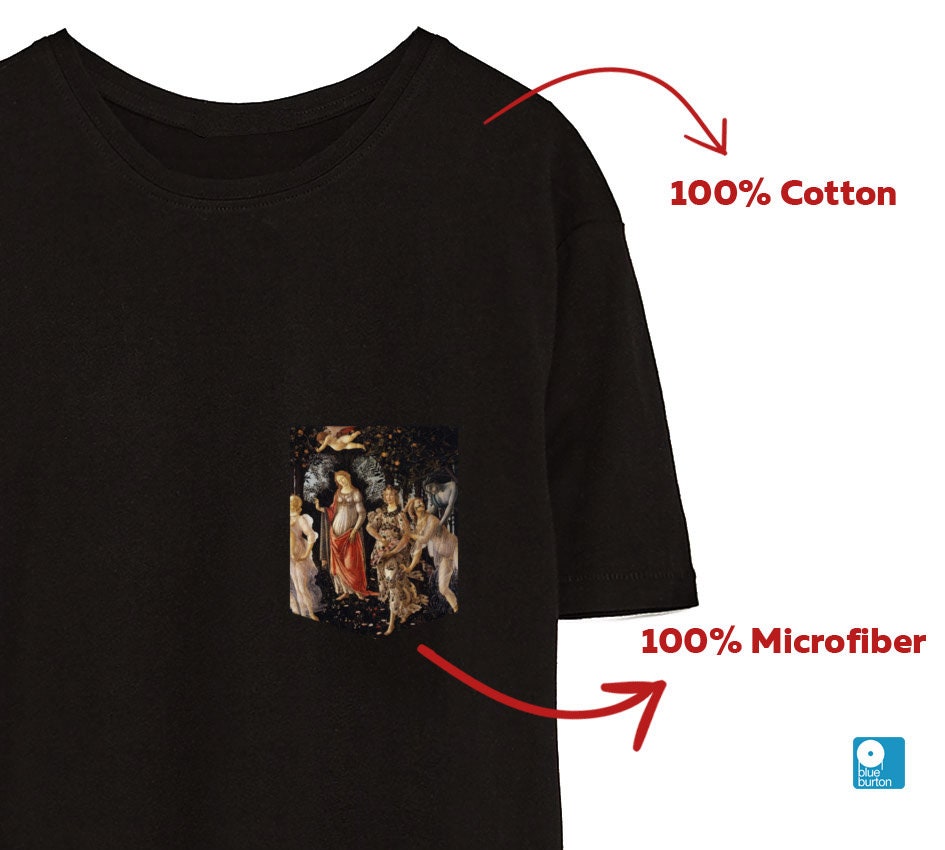This image features a t-shirt displayed against a seamless all-white background. The shirt is oriented with the front side facing the camera and the back side away. The t-shirt's left sleeve is off the frame to the left side. The front side of the collar slightly dips lower than the back side. 

Prominently, the right shoulder of the shirt is adorned with an arrow design; the arrow points down to the right, then angles back up slightly. Below the arrow in bold red font is the text "100% Cotton."

About halfway down and slightly below the chest area on the left side, there is a small picture depicting a religious scene featuring women in vintage dresses, one appearing pregnant, with a cherub floating overhead and a forest background. Beneath this image, another arrow extends to the right and then angles upright once it reaches the white background. Above this arrow, in bold red lettering, are the words "100% Microfiber."

Near the bottom-right corner of the shirt, about an inch away, is a blue square partially covered by a white circle with a blue center. Below this symbol, the word "blue" is inscribed, followed by the word "burton." The bottom hem of the t-shirt extends out of the frame.